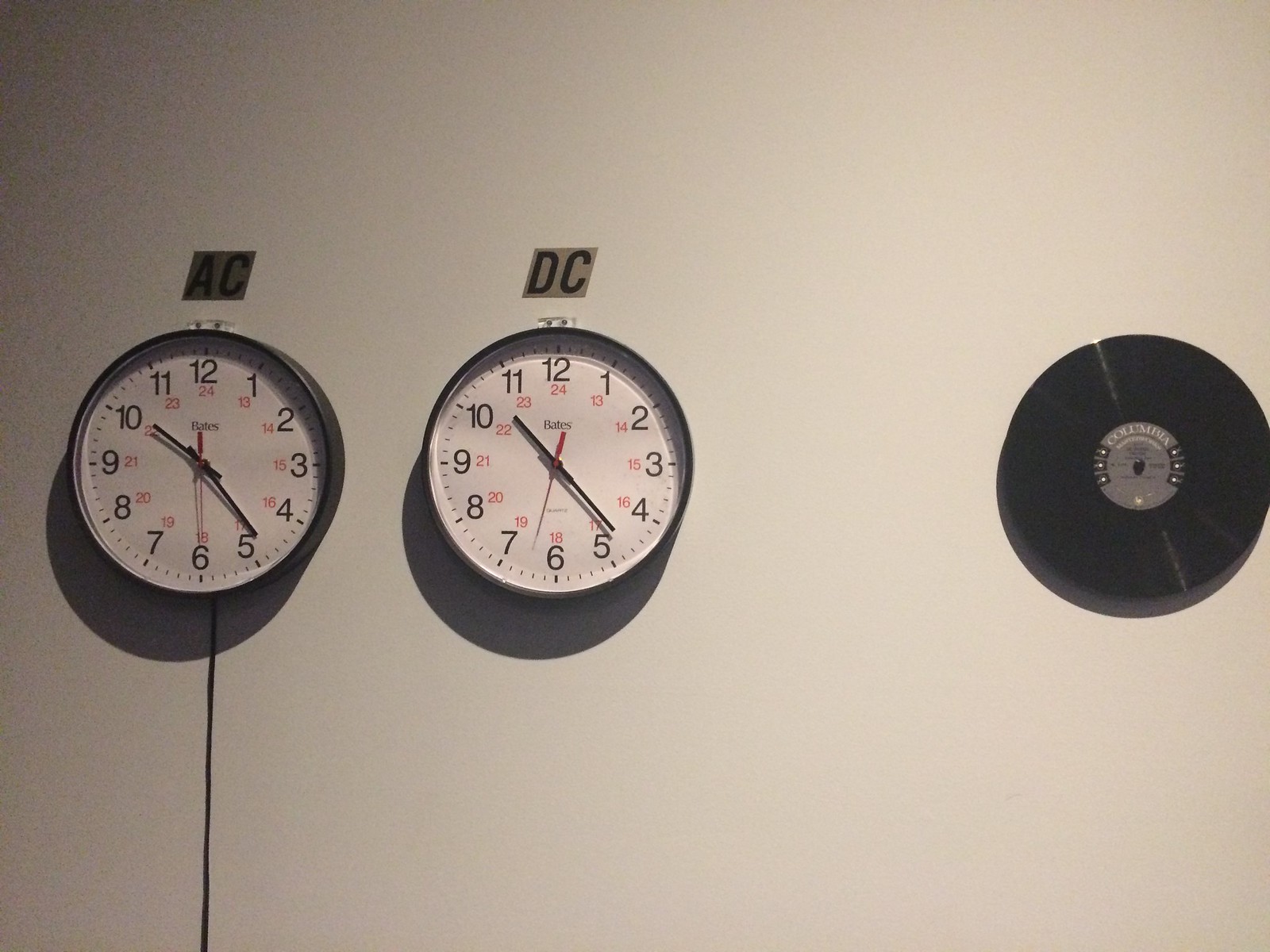The image depicts a well-lit indoor setting with a predominantly white background. Centrally focused yet slightly right-aligned on the wall is a classic black vinyl record, mounted for display. The gray and white label on the record prominently features the brand "Columbia." Surrounding this centerpiece, three black squares with white interiors contribute to the geometric aesthetic of the scene.

To the left of the record, two black clocks hang side by side. Both clocks have white faces, marked with black numerals from 1 to 12, black minute and hour hands, and red second hands. The time on both clocks is approximately 10:23, with the left clock's second hand at 30 seconds and the right clock's second hand at around 33 seconds. An electrical cord extends from the bottom of the left clock, trailing downward.

Above these clocks, gold stickers label them with the letters "AC" for the left clock and "DC" for the right one, contributing to a decorative and thematic element on the white wall.